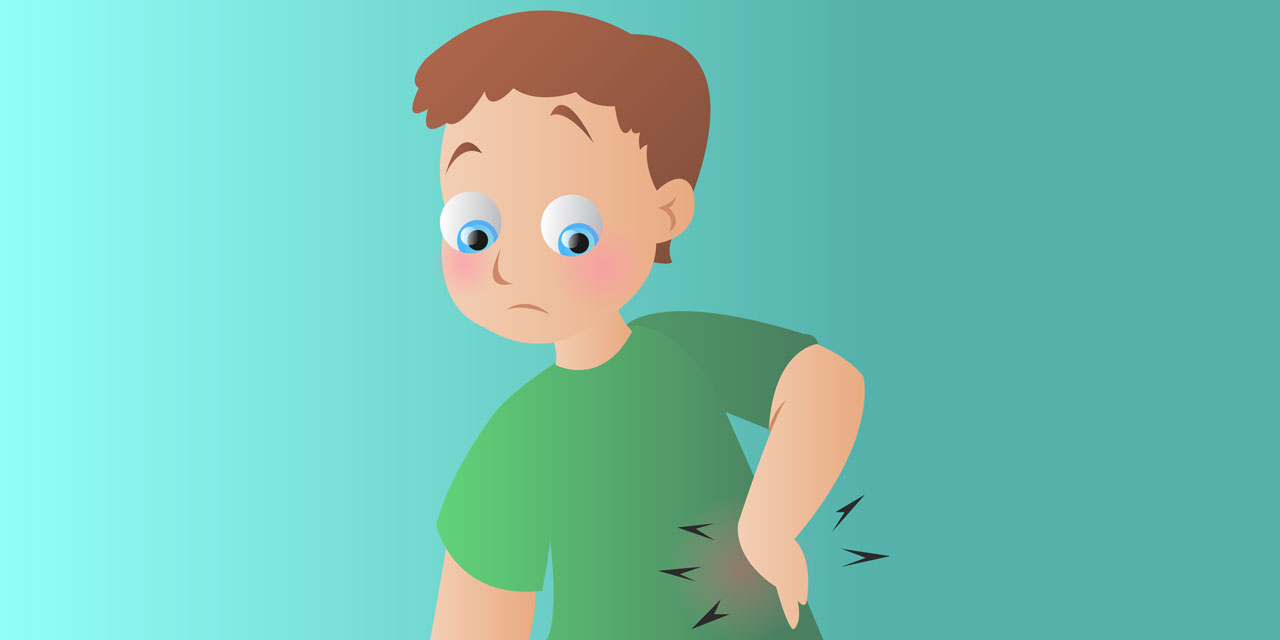In this digital cartoon image, a young boy is depicted from the waist up, wearing a short-sleeved green shirt. His face conveys a sense of sadness, with his blue eyes cast downward and his right eyebrow raised higher than the left, suggesting a troubled expression. His short brown hair frames a face marked by rosy cheeks, highlighted with two distinct pink circles. With one hand placed on his waist, the boy appears to be in discomfort, emphasized by a pink spot at the point of contact and five small triangles radiating outward—three to the left and two to the right. All this is set against a tranquil mint or turquoise blue background, which contrasts with the boy's emotional and physical distress.